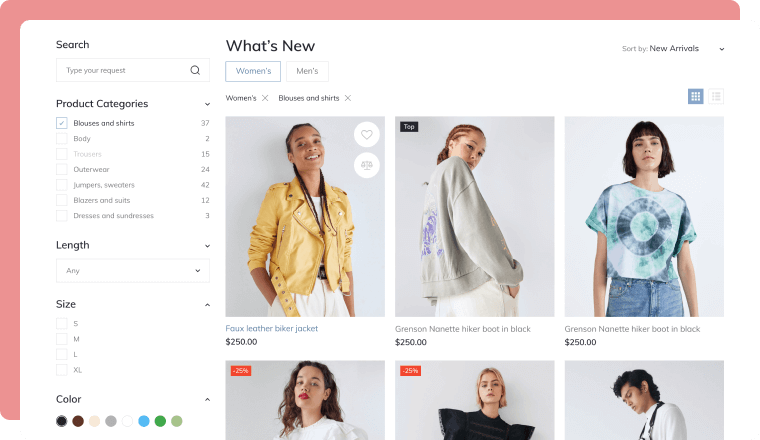The image is a screenshot from an online store's interface. The page features a light peachy pink background border with a white content area. 

At the top, there's a search bar that prompts "Type your request" accompanied by a microscope icon. Just below this, the text "What's New" appears in black, with a highlighted "Women's" button alongside an available "Men's" button. To the right, a sorting option labeled "Sort by New Arrivals" is visible.

A sidebar on the left lists "Product Categories" divided into options such as Blouses and Shirts, Body, Trousers, Outerwear, Jumpers, Sweaters, Blazers and Suits, Dresses, and Sundresses, each accompanied by checkboxes. Below, a "Length" section offers customization options for length and sizes, ranging from Small to Extra Large.

Six clothing item images are displayed in a grid format:
- Top left: A light-skinned Afro-American woman with braids, modeling a yellow faux leather jacket paired with white trousers.
- Top center: A white woman with tightly braided reddish cornrows, wearing a sweatshirt featuring purple graphics, partially turning her head and covering part of her face with her shoulder.
- Top right: A white woman with a blunt bob haircut, dressed in a green and blue tie-dye shirt and jeans.
- Bottom left: A white woman with red lipstick and long brown hair, seen from the shoulders up, wearing a white ruffled blouse.
- Bottom center: A white woman with a blonde bob, wearing a black ruffled dress with a high neckline.
- Bottom right: An androgynous person with short black hair, wearing a white shirt and black suspenders.

Towards the lower left corner, there's a section titled "Color" with square swatches of colors including black, brown, cream, gray, white, turquoise, green, and light green.